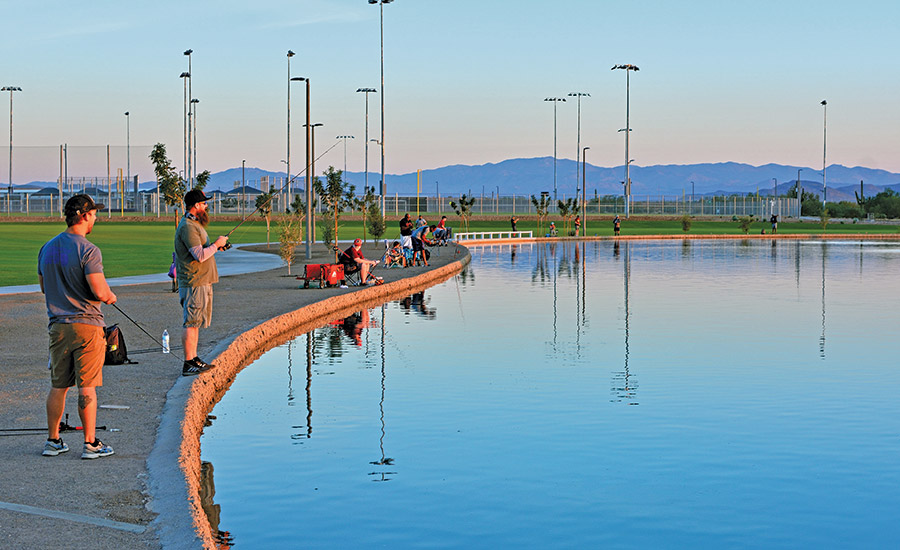The photo depicts an outdoor scene around a large, calm pond in a park, featuring a number of men fishing along a concrete sidewalk. They are dressed in shorts, t-shirts, sneakers, and baseball caps. Some of the men are standing, while others are sitting, casting their lines into the water. The pond is surrounded by green grass and sports fields, enclosed by a chain-link fence. Numerous tall light poles are positioned around the area, illuminating the scene. In the background, there are mountains under a gray sky. The reflections of the light poles create subtle ripples on the pond's surface. One man on the left wears a blue short-sleeve top, orange-brown shorts, and a black baseball hat, with fishing gear in a red canvas wagon nearby. Another man, similarly dressed, is seen with his fishing pole raised, while yet another sits further down with a red hat and wagon.